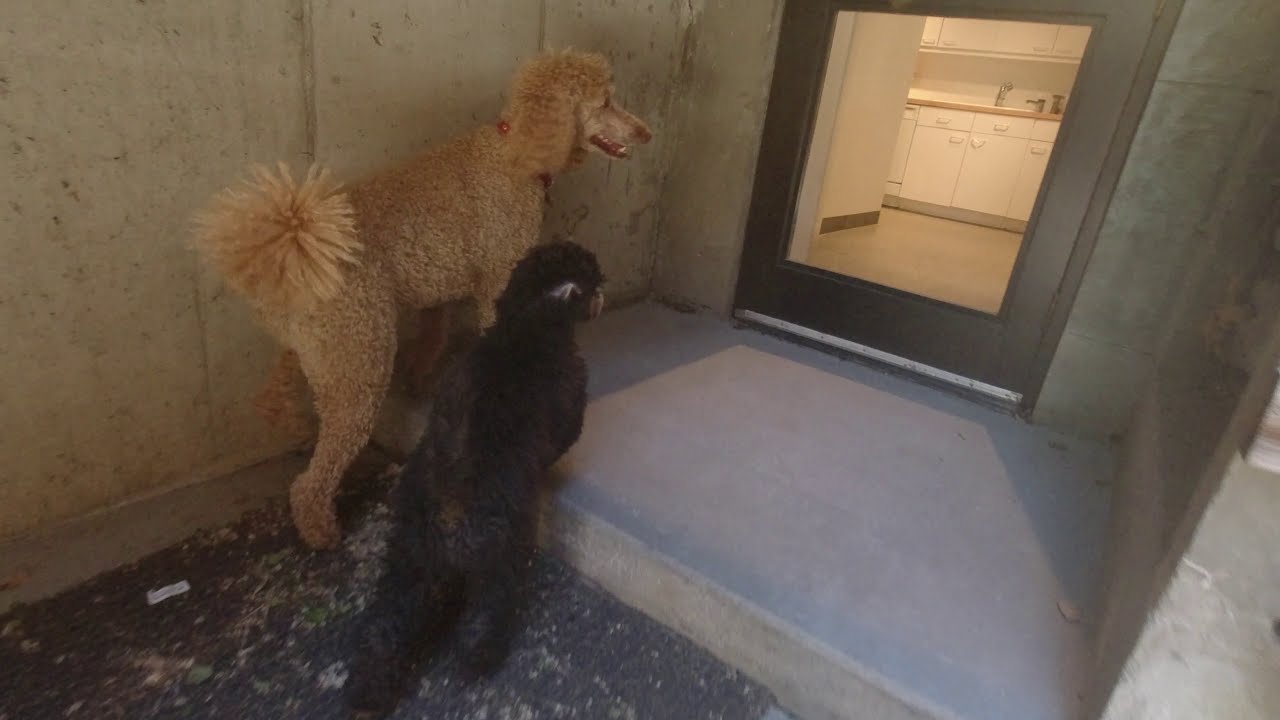In this captivating image, we observe two poodles eagerly awaiting entry through a partially open, glass-paneled door framed in dark gray. Positioned on a concrete step outside the entrance, the larger poodle on the left sports a light brown coat with a distinct, bushy tail, its front paws resting on the step. Beside it stands a smaller black poodle on the right, also with its front feet on the step. Both dogs are intently staring into a well-lit kitchen visible through the glass door, revealing white cabinets, wood-colored countertops, and a light-colored floor with wooden trim. The exterior area around the step features black gravel, and the wall beside the dogs displays a warm yellowish-brown hue.